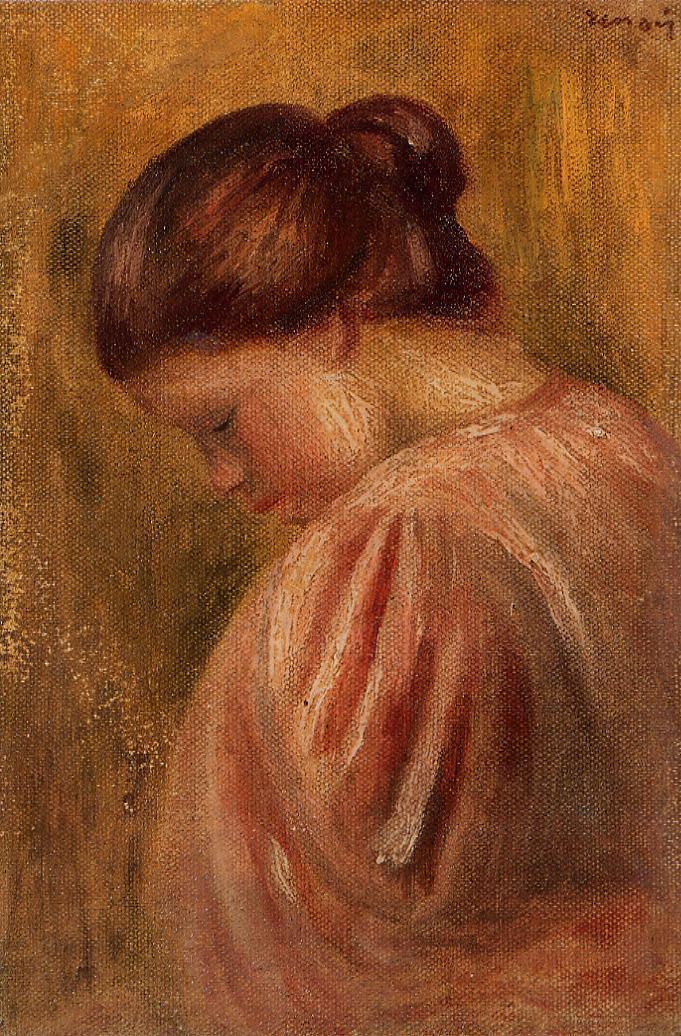This detailed oil painting on textured canvas depicts a young woman in a side profile, positioned against a background with hues of light orange, yellow, and light brown. The woman's chestnut-colored hair is elegantly styled in a bun, and her head is gently tilted downward, conveying a serene and introspective demeanor. Her eyes are closed, accentuated by black eyelashes, and she has delicately pink lips. She is wearing a peach-colored pleated blouse or dress, which appears somewhat amorphous and blends subtly with her form. The background is speckled with white streaks, which also appear on her cheeks and down her neck, adding a sense of depth and dimension. Notably, this atmospheric piece is signed in cursive at the upper right corner, possibly reading "Rimoy" or "S-E-N-A-I-Y," though it is somewhat difficult to decipher. The texture of the canvas itself contributes significantly to the overall aesthetic, highlighted through dotted patterns visible across the painting.